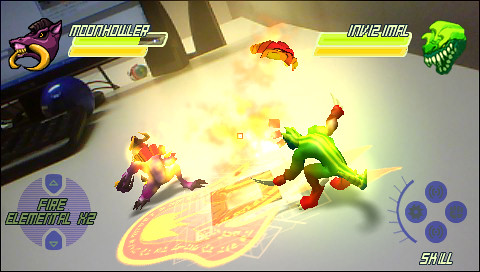In the image, which seems to be a screenshot from a video game, the top left corner displays the name "Moon Howler" along with a partially depleted green health bar and a clear yellow bar. On the left side of the screen, there's a boar-like creature colored purple with striking yellow tusks. Opposite this creature, on the right, the name "Invisi-mon" is shown. Invisi-mon is depicted as a green, alien-like entity with a massive open mouth lined with very large, fang-like teeth. Its health and yellow bars are fully intact.

The center of the image prominently features the green creature, Invisi-mon, which has red hands, feet, and claws on its arms. Meanwhile, the boar-like creature on the left appears to be engulfed in flames and injured, showing a purple hue to its damage.

On the very left side, at the bottom left corner, there is an arrow pointing upwards and another pointing downwards, with blue marks forming a circle in between. The text "Fire" and some elemental labeling follow these symbols.

Towards the right side of the image, a control interface can be seen, with four buttons placed in a circular arrangement: one at the top, one to the right, one at the bottom, and one to the left. Each button has distinct patterns inside. Adjacent to this interface, towards the left, there is an arch with a small line extending from it.

At the very bottom of the image, the word "Skill" is displayed. The scene appears to be set in a location where the floor features a flame-like symbol adorned with red and yellow hues. There seems to be a structure in the top left that resembles a computer, suggesting that the battle may be taking place in a simulated or artificial setting.